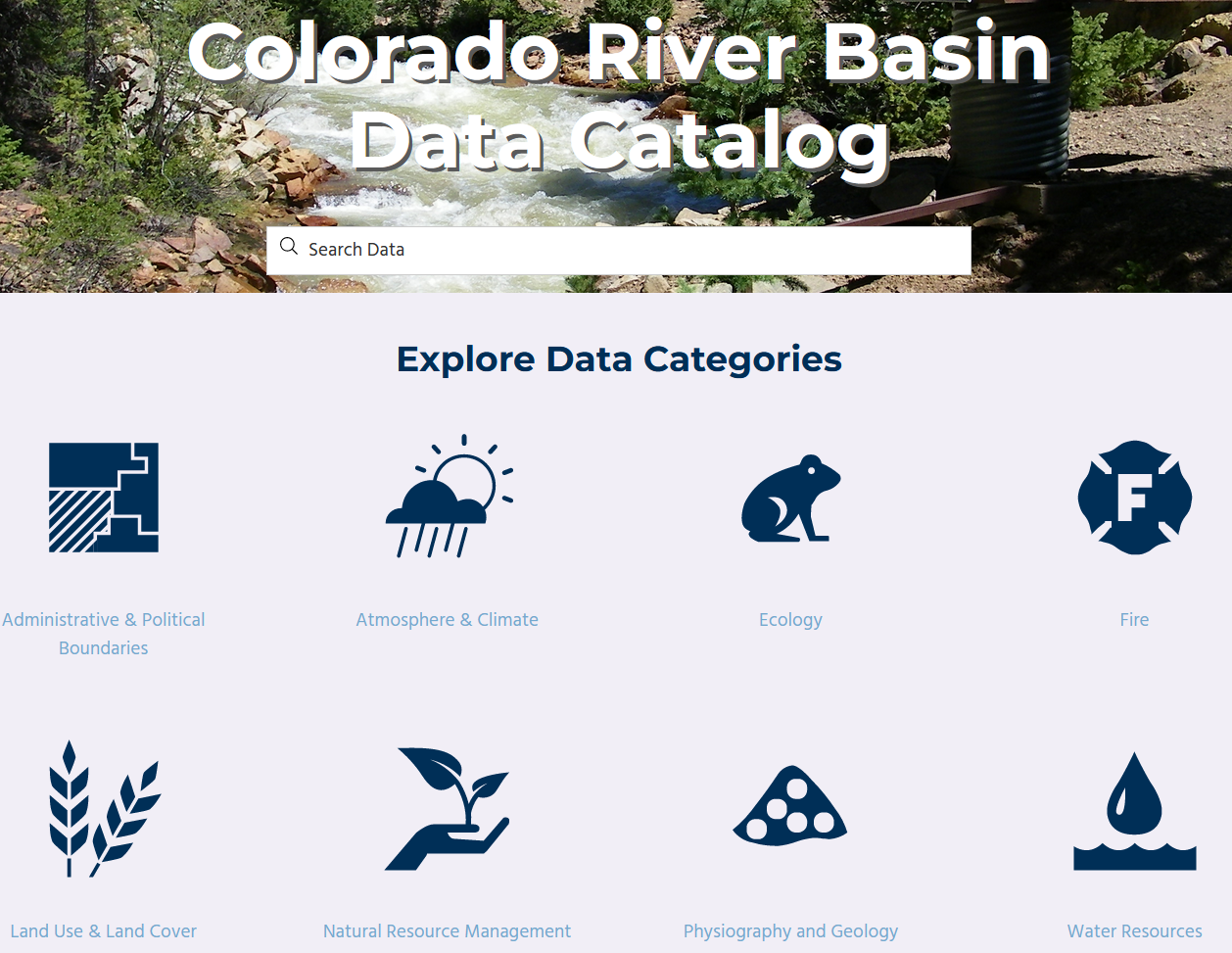The image features a light blue background with a central focus on a picturesque photograph at the top. This photograph showcases the scenic Colorado River flowing serenely, flanked by lush trees, natural rocks, and a prominent trash can, symbolizing both nature's beauty and the importance of maintaining its cleanliness. 

Below this captivating image, bold text announces the "Colorado River Basin Data Catalog," accompanied by a large, inviting search box for users to explore the vast data repository. 

The image further lists eight distinct data categories in a structured layout against the blue backdrop: Administration and Political Boundaries, Atmosphere and Climate, Ecology, Fire, Land Use and Land Cover, Natural Resource Management, Physiography and Geology, and Water Resources. 

This setup emphasizes the extensive and varied data available for exploration within the catalog, encouraging users to delve into specific areas of interest, such as water resources, fire ecology, or atmospheric conditions.